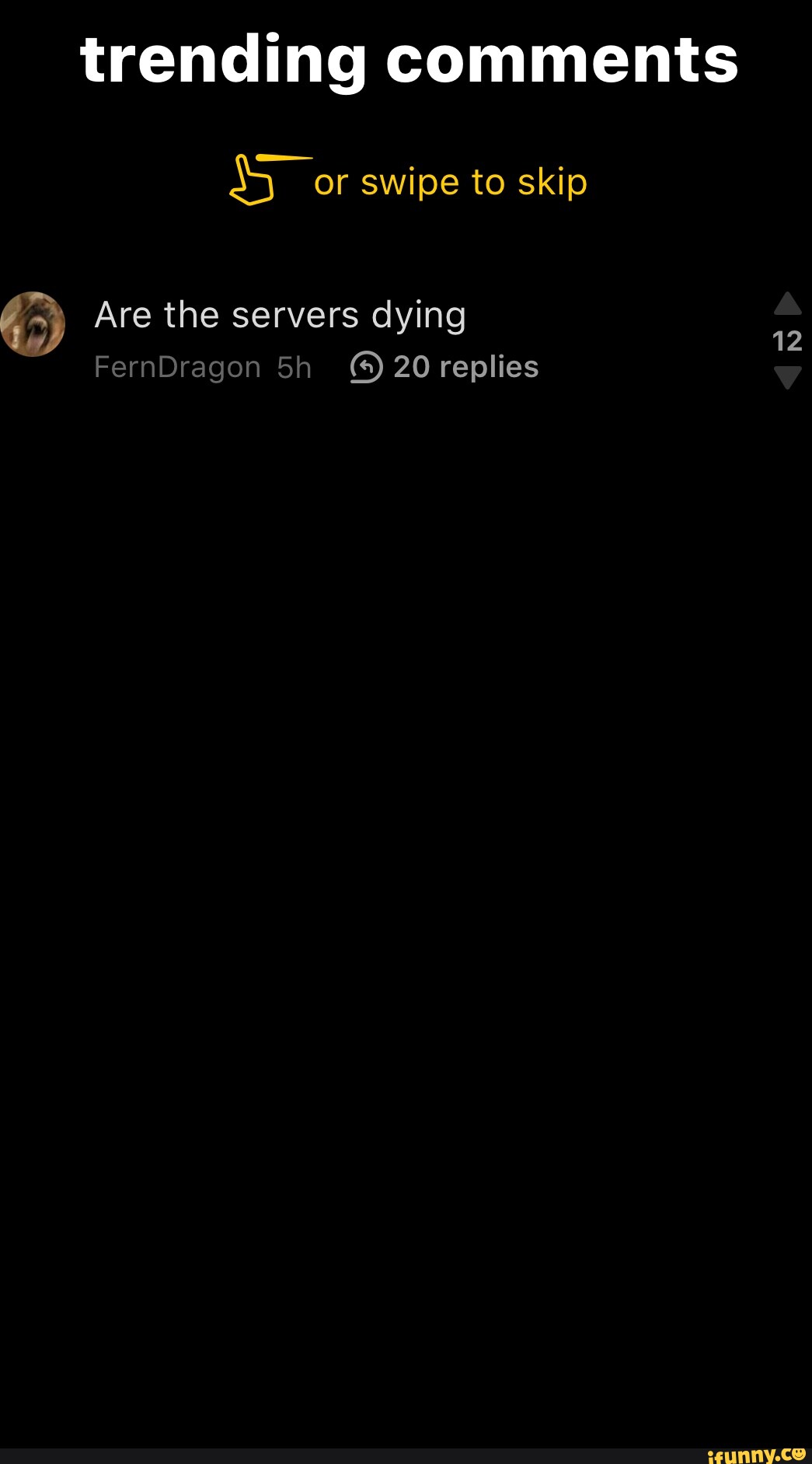The image depicts a cropped screenshot of a social media site with a black background. At the top, bold white text partially reads "Trending Comments," with the rest obscured by cropping. Below this header, there is a gold or yellow hand icon performing a swiping gesture, accompanied by a yellow line and the text "Swipe" or "Swipe to Skip." Directly beneath this, a user's avatar, depicting a dog, is shown with the username "Fern Dragon" in white text. The user's comment, "Are the servers dying?" is also in white, posted five hours ago, and has received 20 replies. On the right side of the comment, an upvote count of 12 is visible. In the bottom corners, the website watermark "ifunny.co" is displayed.